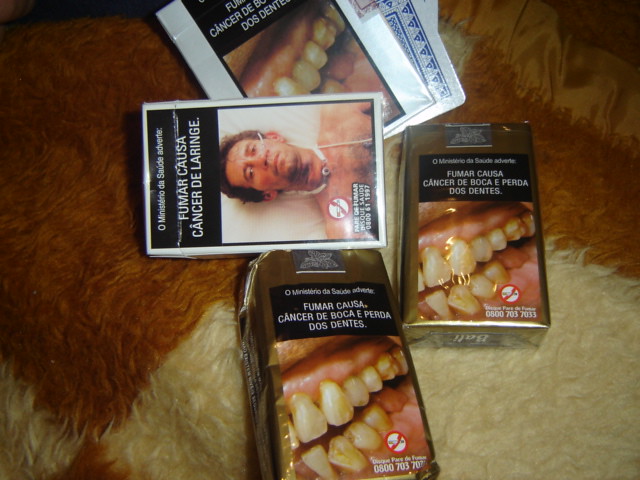This detailed landscape-oriented color photograph captures several gold cigarette packs displayed on a brown and white fuzzy rug, with the rug featuring a gradient from white at the bottom to brown at the top. Nestled among the packs are a few playing cards, partially hidden beneath the central pack. The cigarette packs prominently feature stark warning labels in a foreign language—likely Spanish or Portuguese—emphasizing the severe health risks associated with smoking. The warnings, displayed in a black strip with white text across the top of each pack, include messages such as "Fumar causa cancer de larynx" (smoking causes larynx cancer) and "Fumar causa cancer de boca y perda dos dentes" (smoking causes mouth cancer and tooth loss). These texts are graphically underscored by disturbing color images: one pack shows vivid pictures of decaying and missing teeth, while another portrays a man with a tracheostomy, indicating severe throat surgery necessitated by smoking. This stark and realistic product photograph highlights the dire consequences of smoking through powerful visual and textual warnings.